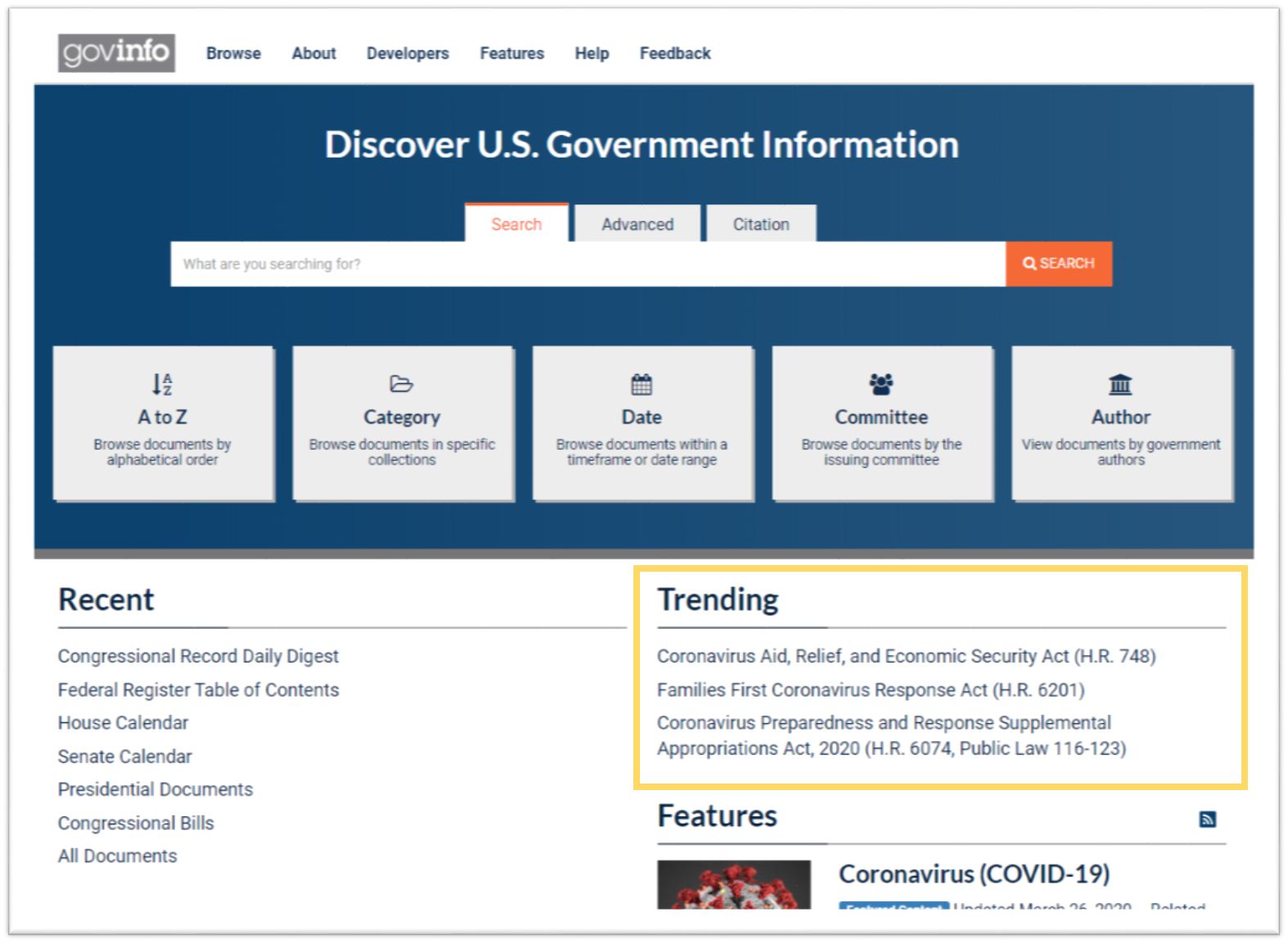This is a detailed screenshot of the GovInfo website, an online platform for accessing U.S. government information. The website features a clean, white background with a blue header at the top. The header includes several navigational tabs in blue: Browse, About, Developers, Features, Help, and Feedback.

The main body of the website is also predominantly blue and prominently displays the text "Discover U.S. Government Information" followed by a large search bar asking, "What are you searching for?" with an accompanying orange search button. Below the search bar, there are three tabs: Search, Advanced, and Citation.

Further down, the website presents five categories represented by large, rectangular gray buttons. These categories are A to Z, Category, Date, Committee, and Author. They are conveniently placed right below the search engine for easy access.

In the lower section of the page, a list of recent documents is displayed. These include the Congressional Record Daily Digest, Federal Register Table of Contents, House Calendar, Senate Calendar, Presidential Documents, Congressional Bills, and All Documents.

To the right of this section, there is an article section labeled "Trending." It lists items such as the Prentice Aid, the Relief and Economic Securities Act, the Coronavirus Response Act, the Coronavirus Preparedness and Response Supplemental Appropriations Act, among others, with additional articles displayed below.

The design and layout of the website facilitate user navigation and access to a wide range of government information.